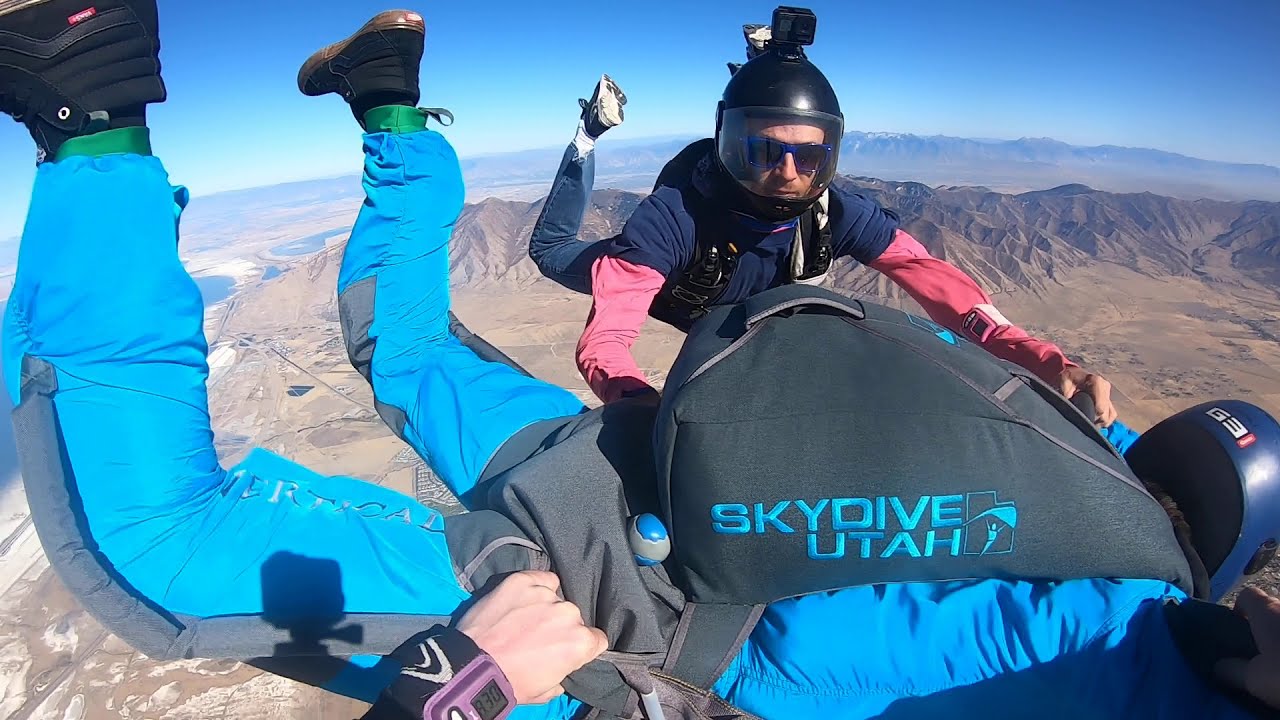The image captures three skydivers in action over a mountainous, partially desert-like area in Utah. The central figure, equipped with a Skydive Utah parachute and helmet, is wearing a light blue jumpsuit. Two other skydivers are grasping him; one has a camera mounted on a black helmet and is sporting a red and black outfit with distinct blue sunglasses, pink long sleeves, a blue jacket, and blue jeans. The photo appears to be taken from the perspective of the person on the left, whose left hand is visible gripping the central skydiver. This individual is wearing a purple watch on their wrist. The mountainous backdrop features not only rugged terrain but also glimpses of residential areas and lakes. The dynamic aerial shot vividly conveys the thrill and precision of the skydivers' coordinated maneuvers.